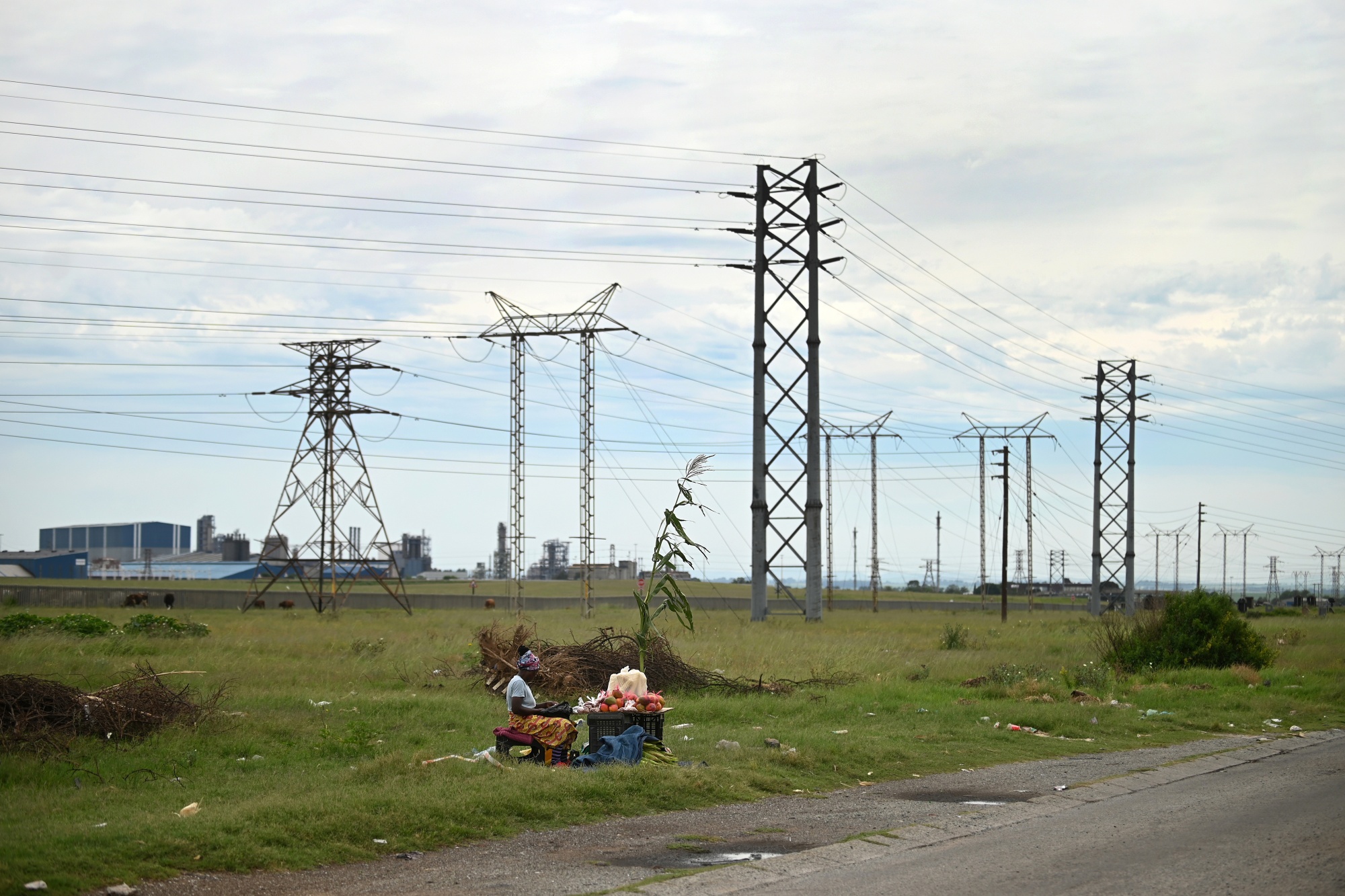The photograph captures a scene by the roadside, featuring a grassy area littered with trash. An individual, likely a black woman, is seated on a chair near the edge of the paved road. She's wearing a purple bandana, a light blue short-sleeved shirt, and an orange skirt. In front of her is a small table displaying what appears to be small pumpkins or orange and red fruits, and several dark blue and green blankets are spread out on the ground in front of the table. 

The road, visible in the lower right corner, has a couple of puddles and gravel patches. The grassy field, dotted with brown and green bushes, extends beyond the road and shows evidence of litter, including an overflowing trash bin. 

In the distance, a series of high-voltage power lines stretch across the sky, supported by large metallic towers. Farther back, on the left-hand side of the image, a structure resembling a coal plant is visible, with additional buildings scattered in the background. The sky above is mostly overcast with white and gray clouds, creating a somber atmosphere.